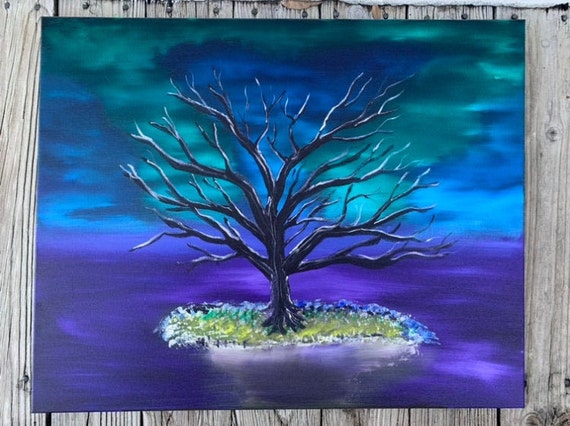A visually striking square art print is set against a backdrop of rustic, weathered wooden boards with visible nails. The gray-brown vertical planks form a rough, aged surface reminiscent of a dock or fence. Centrally positioned on this wooden platform is a rectangular canvas, which appears to be painted with acrylics. The painting itself is a mesmerizing blend of dark colors, featuring a small, oval-shaped landmass surrounded by water. The water transitions from deep blue to shades of purple and light purple. At the center of this tiny island stands a solitary, bare tree with a short trunk and upward-pointing branches, intricately detailed in black with white accents. The sky above is equally captivating, a mix of medium to dark blue, charcoal, and hints of teal and green, adding to the painting's moody ambiance.